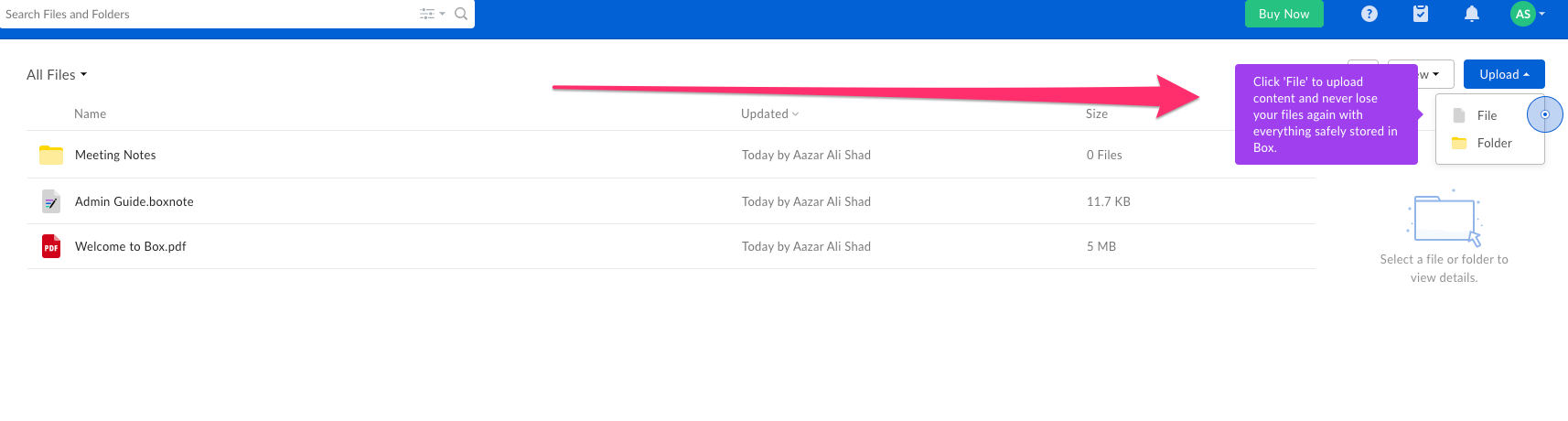This image showcases a wide, horizontally elongated interface with a predominantly white background, except for a medium blue title bar at the top. On the left side of this title bar, there is a search box with a white background and the placeholder text "Search files and folders"; a magnifying glass icon is positioned on its right end. This search box extends approximately one-third of the way across the image. 

In the upper right corner of the title bar, there is a green "Buy Now" button. Adjacent to it, there are multiple icons: a question mark, a check mark inside a box, and a bell. Additionally, in the upper right corner, there is a green circle with the white initials "AS" inside it.

Below the title bar, the main area features a heading in the upper left corner that reads "All Files" in black text. The background here is also white. The content is organized into three columns labeled "Name," "Updated," and "Size" from left to right. Under these columns, there are three items listed: "Marketing Notes," "Admin Guide" (though the last word is not fully readable), and a PDF file labeled "Welcome to [unreadable] .pdf".

The detailed layout and elements of the image suggest a user interface or dashboard, possibly for file management or cloud storage.